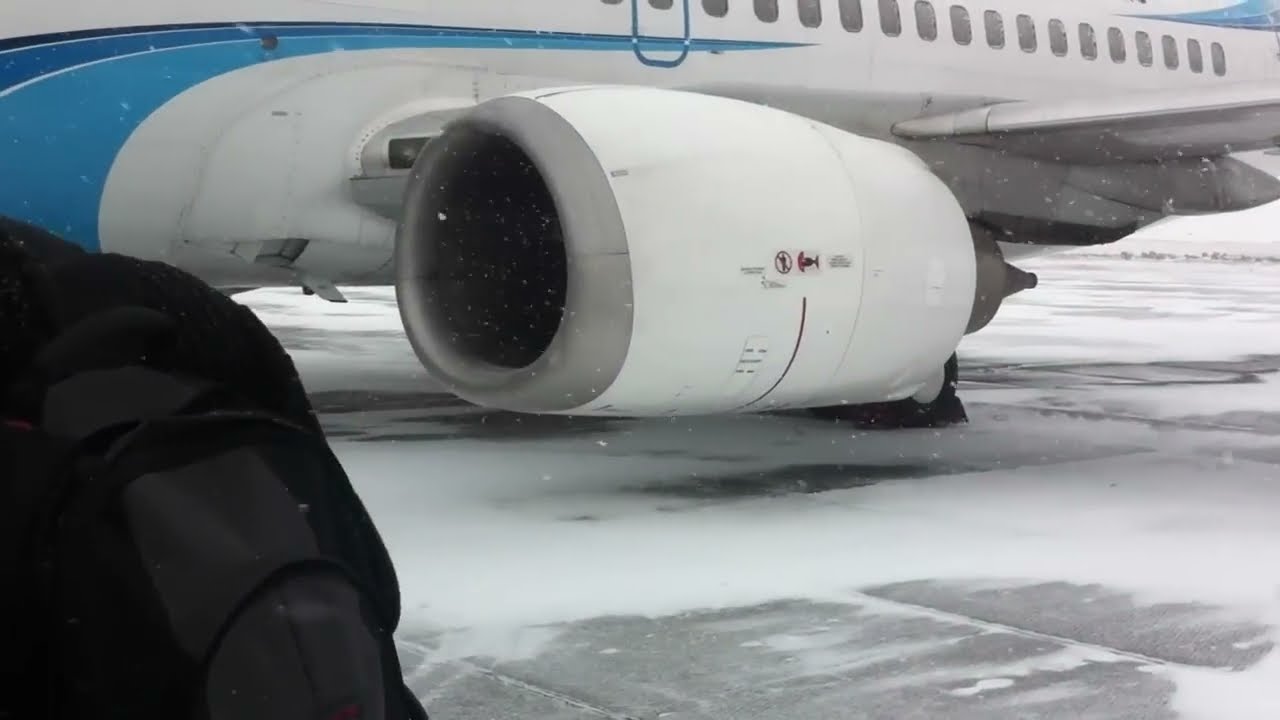In this outdoor photograph taken on a snowy day, the focus is on a large white passenger airplane with both light and dark blue curved designs. The prominent feature in the image is the airplane's turbine, which is clearly in focus and displays a white and gray exterior. Situated on a snow-covered tarmac, the scene also includes a person in a black winter coat with a black backpack standing to the left side of the image, their face not visible. The background consists of a snowy runway and an indistinct white sky, enhancing the wintry atmosphere. The snow on the ground has patchy areas where it has been blown away, adding to the scene's overall detail and texture.